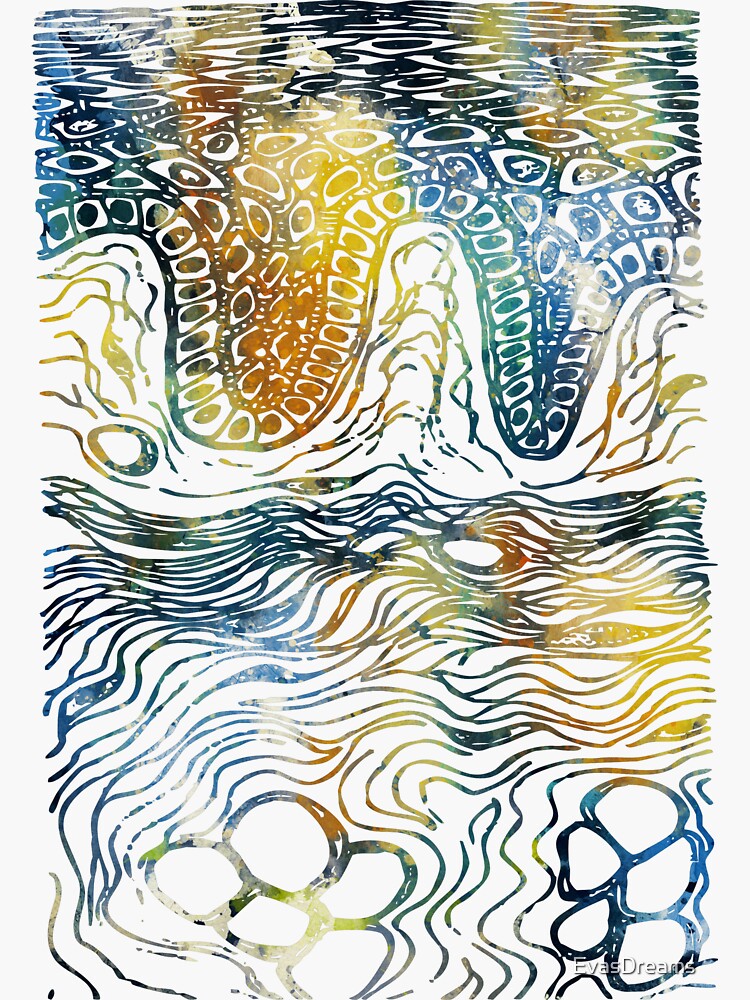This detailed abstract painting features a variety of colorful, intertwined shapes and lines set against a white background. Dominated by a complex array of squiggly lines and geometric forms, the composition includes a range of hues, predominantly blue, brown, tan, black, and light brown, but also features orange, yellow, green, and silver, creating a rainbow-like gradient. The painting is sectioned by different motifs: at the top, there are scale-like designs reminiscent of snake scales that curve gracefully, resembling a wave. Below this, the squiggly lines follow a similar curvilinear motion, with clusters that evoke the appearance of spaghetti strands, intersecting and flowing horizontally. Among these dynamic patterns, circular shapes emerge, some encased in square outlines, with a notable element resembling a flower with round petals and a central round middle, although it is predominantly composed of intricate linework. The painting is watermarked in the bottom right corner with "Ava's Dreams," likely indicating the artist. The piece exudes movement and complexity, drawing the eye with its vivid interplay of shapes and colors.